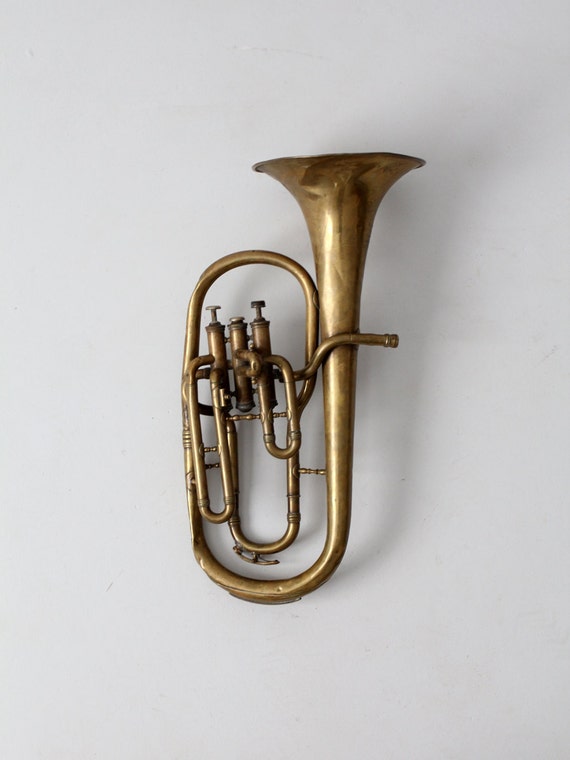A tarnished brass horn, possibly a couple of hundred years old, is mounted against a gray-and-white wall, bathed in soft light. The horn features a large bell that faces upward and gradually narrows, weaving through a series of intricate loops and bends that resemble a paper clip. Central to the instrument are three vertical valves: two are raised, and one is pressed down. A small tube extends horizontally across the horn, leading to the mouthpiece, which is directed to the right. The detailed curves and overlapping loops of the horn showcase its complex design.